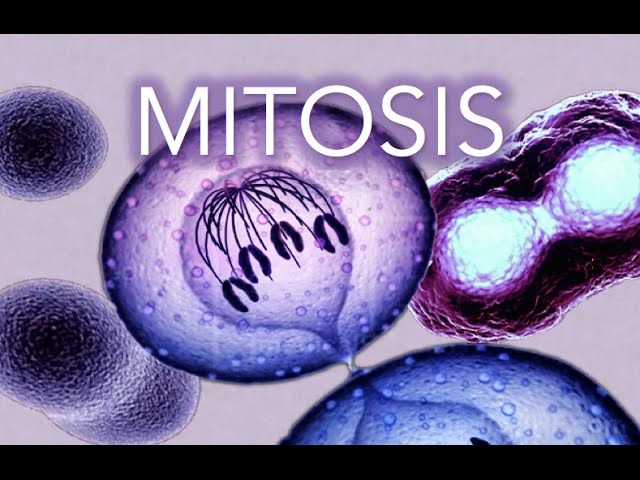This image is a screen capture from an instructional video on mitosis, prominently titled with large white letters "Mitosis" across the top. The background is predominantly purple, featuring an array of cells of varying sizes and consistencies. Encasing the graphic are thick black borders at both the top and bottom.

In the center foreground is a large purple cell adorned with purple dots and displaying what appears to be chromosomes—depicted as black lines with kidney bean-like structures at the ends. This primary cell seems to interact with another partially visible blue cell above it, characterized by blue dots.

To the right, there is a darker purple cell that houses a pair of interconnected structures, resembling embedded eyes. Nearby cells in this region are white with pink outlines. Moving leftward, the cells vary in appearance: one resembles a double-cell formation with dark blue centers and lighter blue peripheries, while another cell, described as looking like a pair of purple oranges or circular bulbs, exhibits dark purple fringes and a black-rimmed boundary. Within these fringed cells, smaller ovals in aqua blue and other shades of purple can be seen.

Overall, the image captures various stages and forms of cells involved in the process of mitosis, set against a visually striking purple backdrop with notable black bordering.